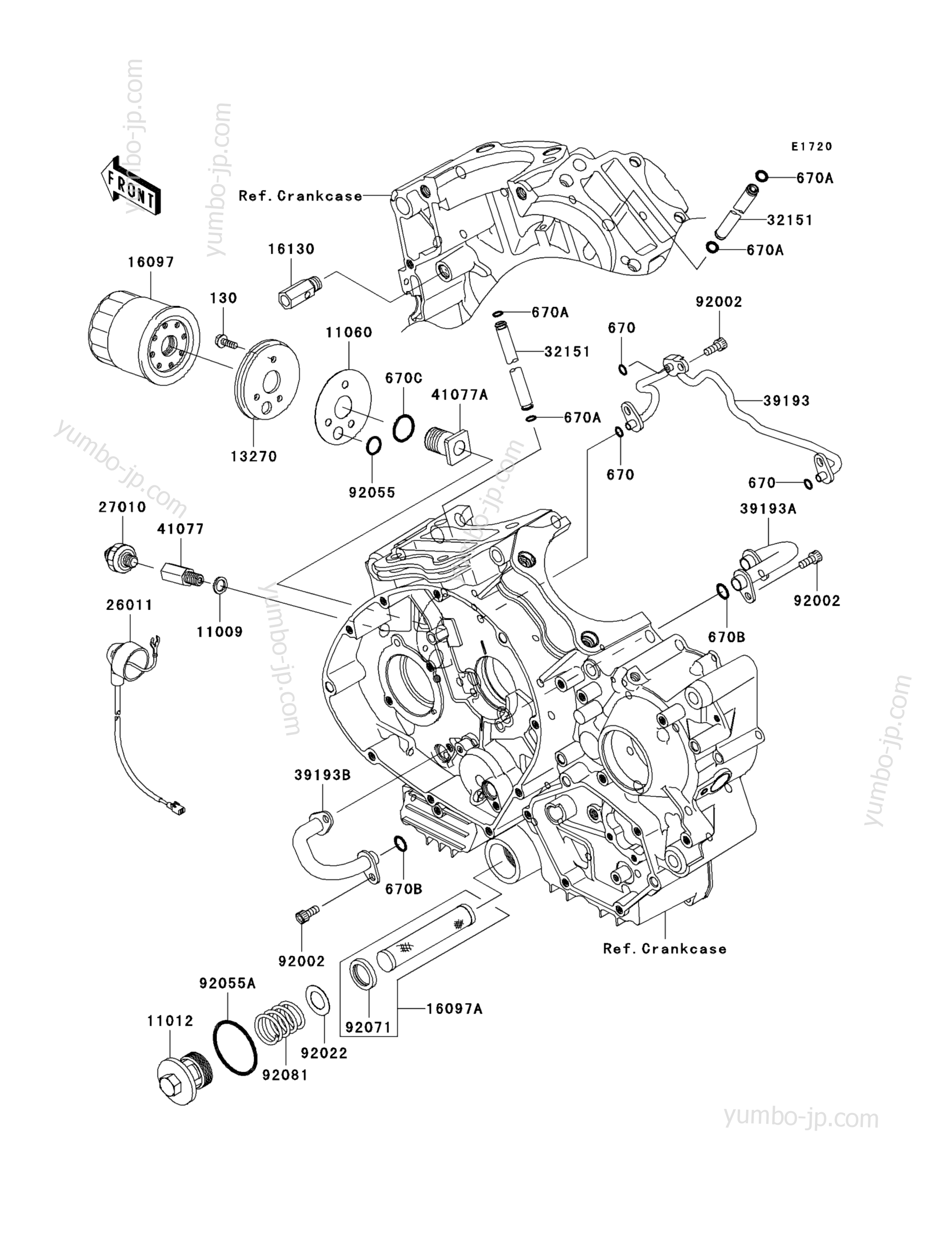The image is a detailed, black and white exploded diagram of an engine, meticulously breaking down every component. Each part is annotated with individual numbers, making it easy to identify screws, pipes, springs, and other components that constitute the engine. Central to the diagram, there's a prominent crankcase with various parts radiating outward, carefully spaced. Instructions and numbers are abundantly present, particularly 1, 1, 0, 1, 2, guiding the assembly process. On the upper right corner, an arrow labeled "front" points to the left, aiding orientation. The entire diagram is set against a stark white background with the website name "yumbo.jp.com" watermarked throughout, adding a unique and professional touch.